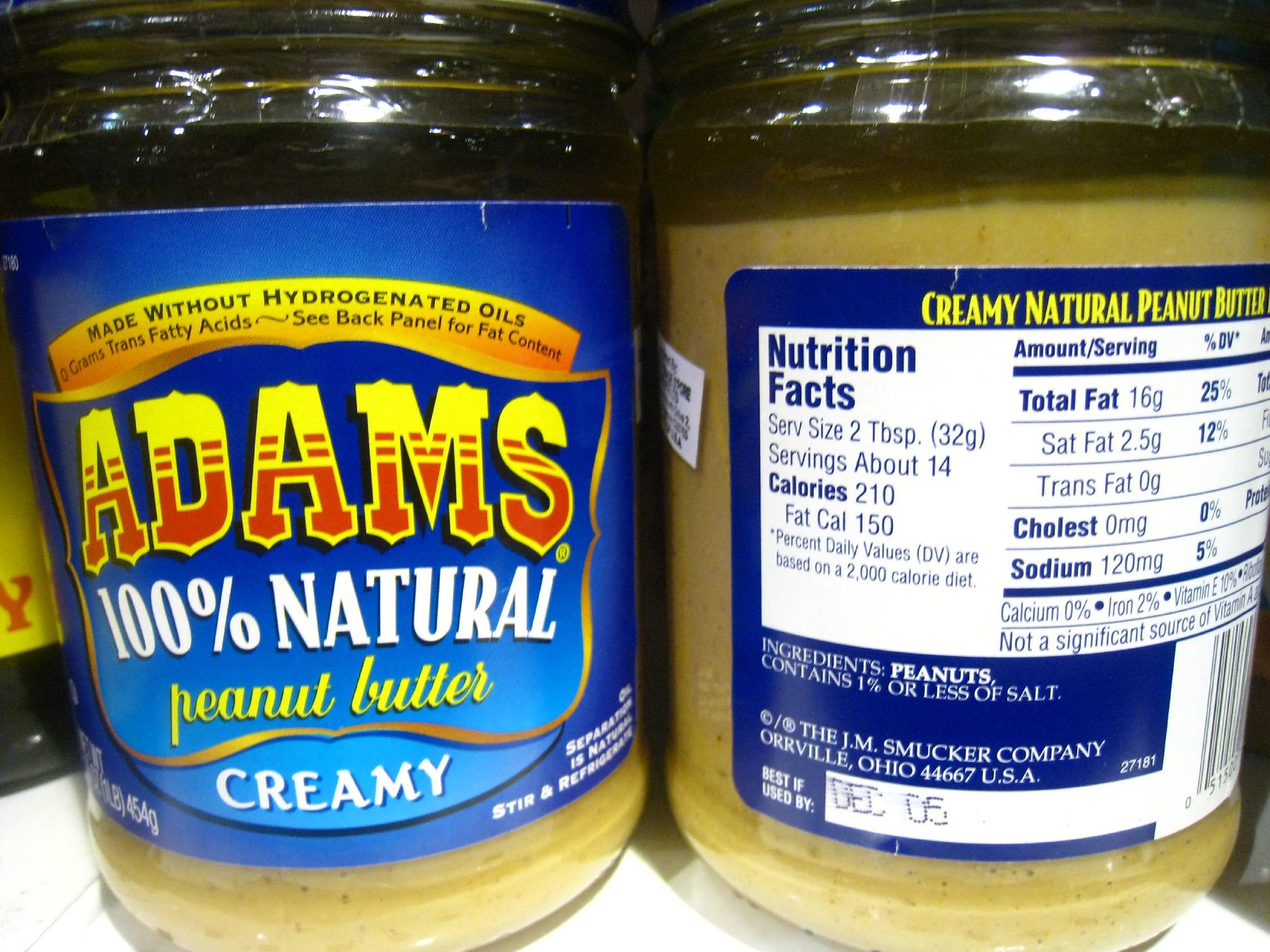The image showcases two glass jars of Adams 100% Natural Creamy Peanut Butter, positioned side by side. The jar on the left provides a full view of the front label, which prominently features the Adams brand name. A bright yellow banner at the top signifies that the peanut butter is made without hydrogenated oils and contains zero grams of trans fatty acids, directing viewers to the back panel for further fat content details. The natural, creamy peanut butter is visible through the transparent glass, adding to the product's wholesome appeal.

The jar on the right mirrors the left one but displays the back label, highlighting the nutritional information. Key details include a serving size of two tablespoons, approximately 14 servings per container, with each serving containing 210 calories, 150 of which are from fat. The total fat content is 16 grams, including 2.5 grams of saturated fat and zero grams of trans fat. There is no cholesterol and the product contains 120 milligrams of sodium. The ingredients list is straightforward, primarily comprising peanuts with 1% or less of salt. At the bottom of the back label, the manufacturer's information is presented: The J.M. Smucker Company, Orville, Ohio 44667, USA. The product's best-by date is clearly marked as December 5th.

This detailed and well-composed presentation of the jars gives potential buyers a thorough understanding of the product's nutritional value and brand reliability.